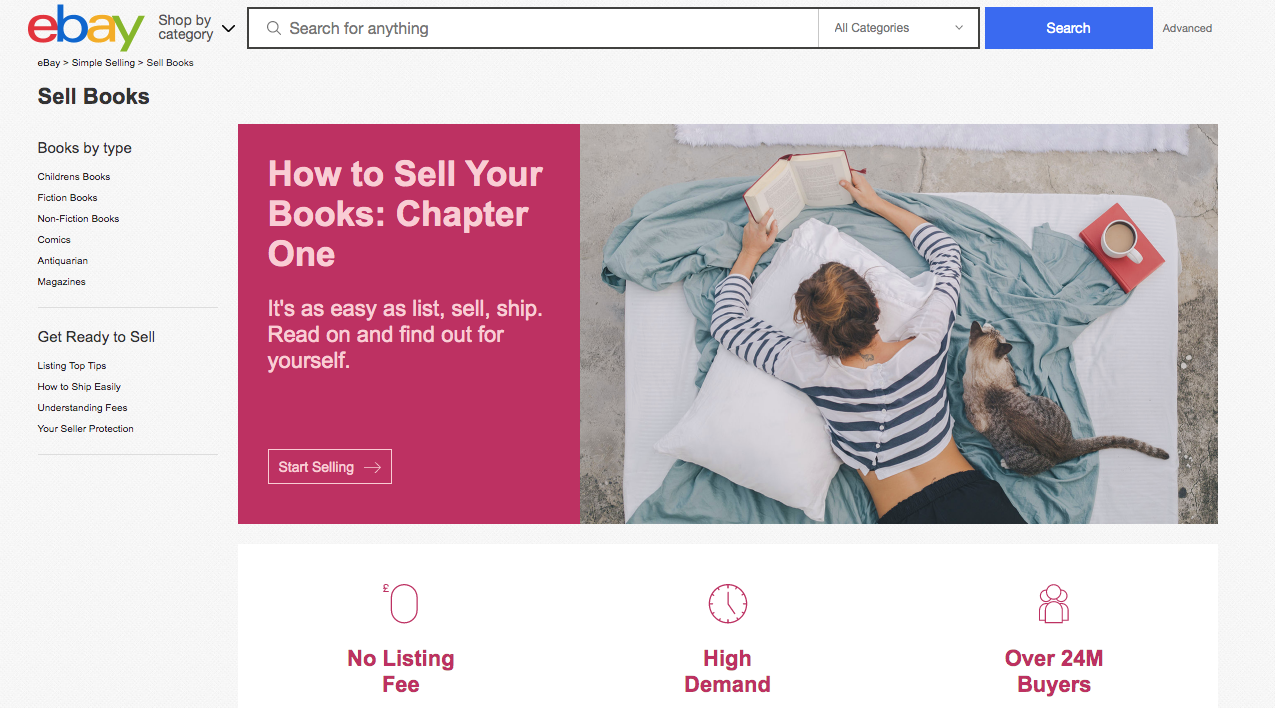The image is a screen capture of an eBay webpage displayed on a desktop. The webpage has a predominantly white background. Dominating the center of the page is a large, detailed picture. To the left side of the screen, a vertical sidebar is visible, featuring the colorful eBay logo at the top. The logo consists of the letters: 'e' in red, 'b' in blue, 'a' in yellow, and 'y' in light green. Directly below the logo, the words "Sell Books" are written in black.

The central image showcases a top-view photograph of a person lounging on a bed while reading a book. A cat, identifiable by its long gray tail, is resting beside the person. The bed is adorned with white and light blue sheets, creating a relaxing backdrop for the scene. On the left side of the image, a pink text box contains the phrase, "How to Sell Your Books: Chapter One," providing context to the eBay listing or article displayed on the screen.